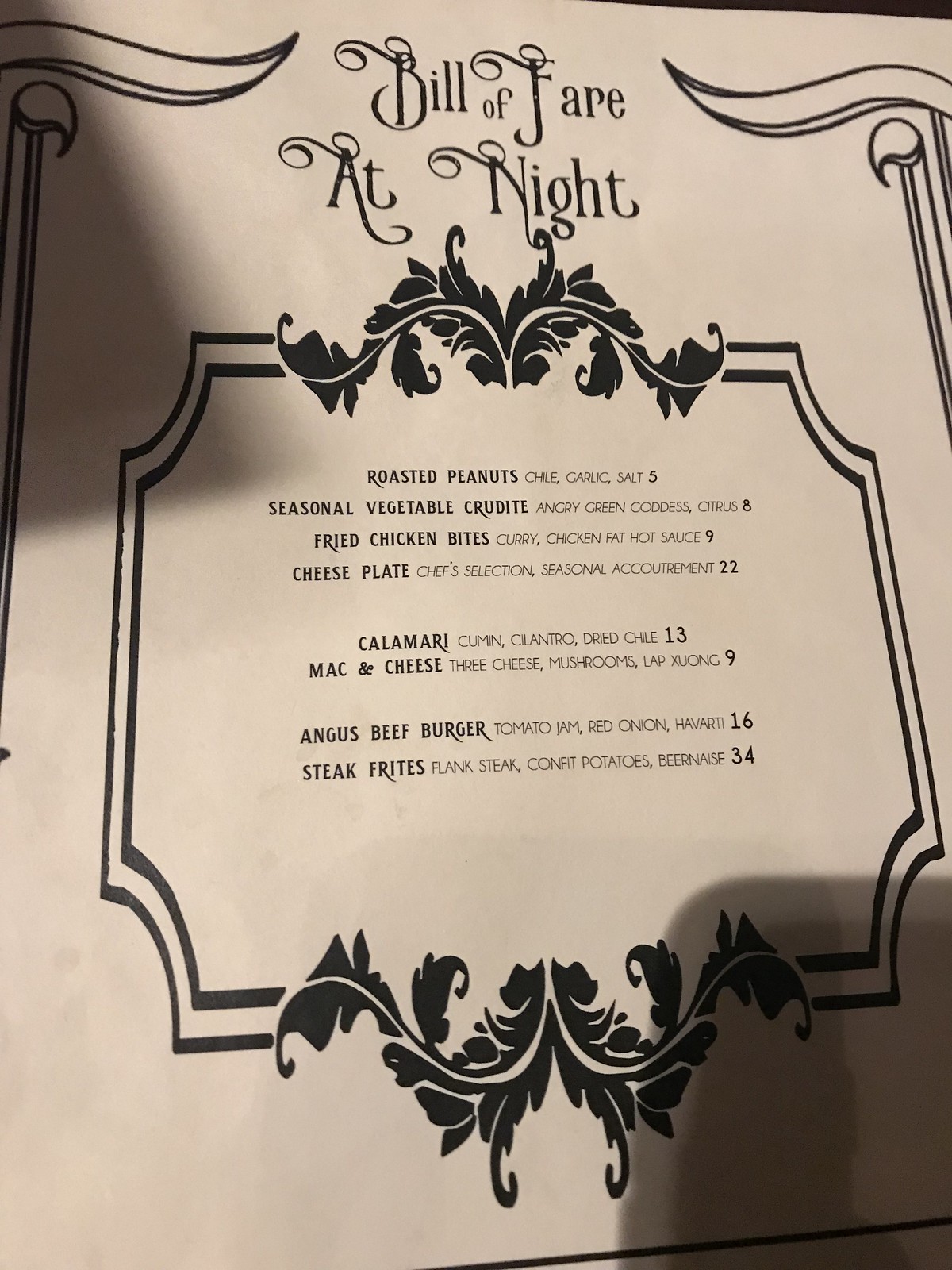The image depicts an elegantly designed restaurant menu titled "Bill of Fare at Night." The menu features a variety of carefully curated items, each detailed with accompanying ingredients and prices. The list includes:

- Roasted Peanuts: seasoned with chili, garlic, and salt, priced at $5.
- Seasonal Vegetable Crudité: served with an 'angry' green goddess dressing and a hint of citrus, priced at $8.
- Fried Chicken Bites: enriched with curry, chicken fat, and hot sauce, priced at $9.
- Cheese Plate: a selection curated by the chef, paired with seasonal accoutrements, priced at $22.
- Calamari: flavored with cumin, cilantro, and dried chili, priced at $13.
- Mac and Cheese: featuring three types of cheese, mushrooms, and lap shuang, priced at $9.
- Angus Beef Burger: topped with tomato jam, red onion, and Havarti cheese, priced at $16.
- Steak Frites: consisting of flank steak, confit potatoes, and béarnaise sauce, priced at $34.

The menu is embellished with intricate margins featuring mistletoe-like designs in black ink. The off-white backdrop highlights the finely detailed menu items. Adding to its sophistication, ornamental pillars frame the left and right sides of the menu. The heading, "Bill of Fare at Night," is presented in an elegant, decorative font, underscoring the refined presentation of the menu.